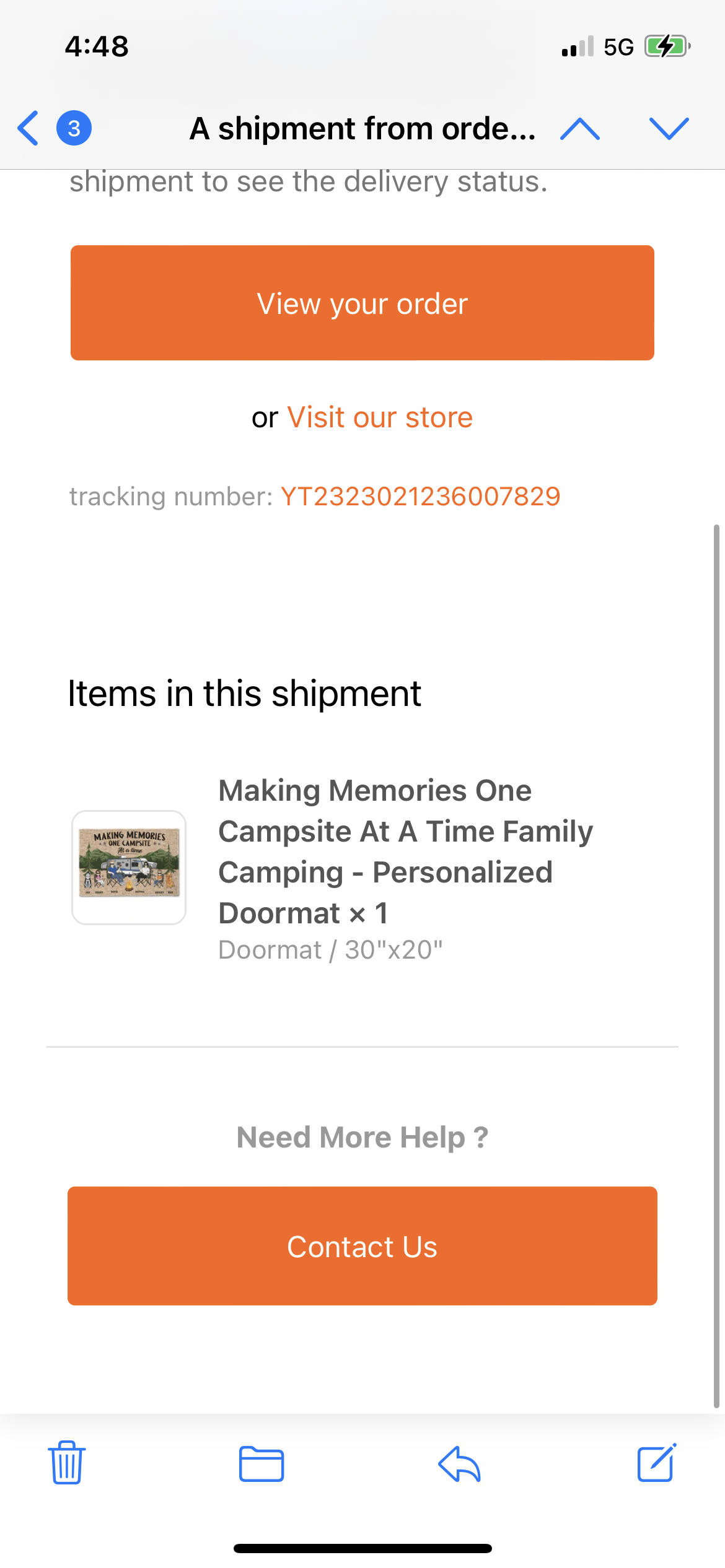The image is a screenshot from a smartphone. On the top left corner, there is a timer displaying "4:48", next to which is a green page icon indicating charging. The smartphone is connected to the NetEck 5G network, represented with a NetEck signal icon.

The open page shows details of a shipment order. It reads, "A shipment from order" and prompts the user to "see the delivery status." An orange button with white text is displayed, labeled "View Your Order."

Further down, the page mentions "Visit our store" in orange text, accompanied by a tracking number, YT2323021236007829, also in orange. The rest of the text is in black, providing details about the items in the shipment: "Making memories one composite at a time. Family camping. Analyze doormat times one. Doormat 30 inches times 20 inches."

On the left side of the main text, there is an image of the doormat, further labeled with "Making memories one composite at a time. Family camping." At the bottom of the page, it says "Need more help?" followed by an orange button labeled "Contact Us."

There are several blue icons at the bottom of the screen for various actions, starting with "Delete" on the bottom left, followed by "File" and "Share", and ending with another icon on the bottom right.